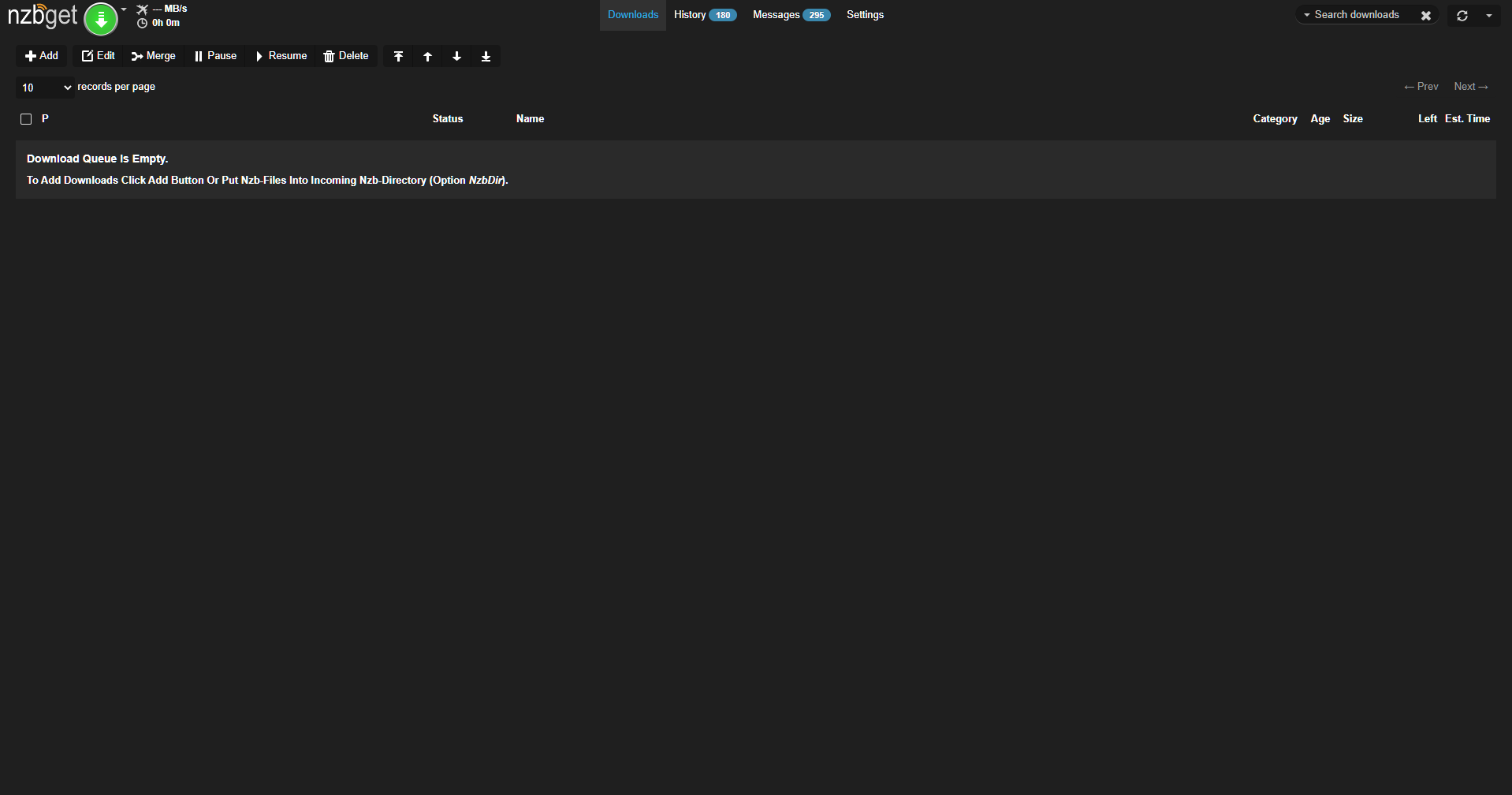The image is a screenshot of a webpage with a completely black background. At the top left corner, the text "NZBGET" is prominently displayed next to a green circular logo featuring a white arrow pointing downwards. To the right of this logo, two small, white options are visible but their labels are not clear due to their size. 

In the center of the page, three main categories are organized horizontally: "Home" accompanied by a round blue icon, "Messages" with a similar blue icon, and "Settings" written in white text. On the furthest right, standard webpage control options for minimize, refresh, and close (X button) are visible.

Directly below the "NZBGET" logo, a small panel contains several options such as "Merge," "Add," and other functionalities written in very small white font. The top of the webpage features a banner with very small and unreadable white text. To the right of this banner, partially legible labels such as "Company" and "Age" appear, followed by other indistinguishable words due to the tiny text size.

A light black banner spans the entire width of the page, displaying white lettering that remains unreadable even upon close inspection.